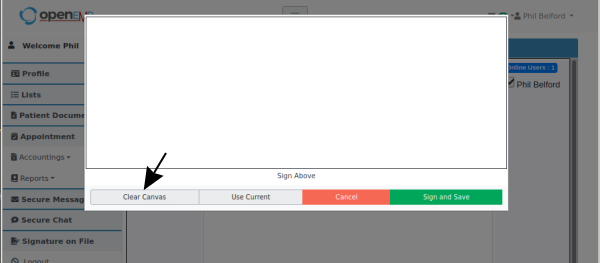The image features a user interface pop-up. The background is gray, likely modified from its original white color due to the pop-up overlay. Within the background, there's a light blue circular element with black, underlined text that reads "open end." Notably, the letters "E" and "D" in "end" are highlighted in blue.

On the right side of the interface, there is a silhouette of a person labeled "Phil Belford." On the left side, in bold black text, it reads "Welcome, Phil." Below this, there are truncated words "Profile with patent documen...", indicating the rest of the document text is cut off. Additional options listed include "Appointment," "Accountings reports" in gray, "Secure message" (with the 'E' cut off), "Secure chat," and "Signature on file."

The pop-up window itself features a white interior with a gray border. The majority of the pop-up, specifically the top three-fourths, is blank. At the bottom center of this window, gray text instructs "Sign above," with a black arrow pointing towards a button labeled "Clear canvases" in gray text on a gray background. Additional options include "Cancel" in white text on an orange background, and "Sign and save" in white text on a green background. 

The interface appears cluttered yet straightforward, providing various instructions and options for user interaction, specifically for the individual named Phil Belford.